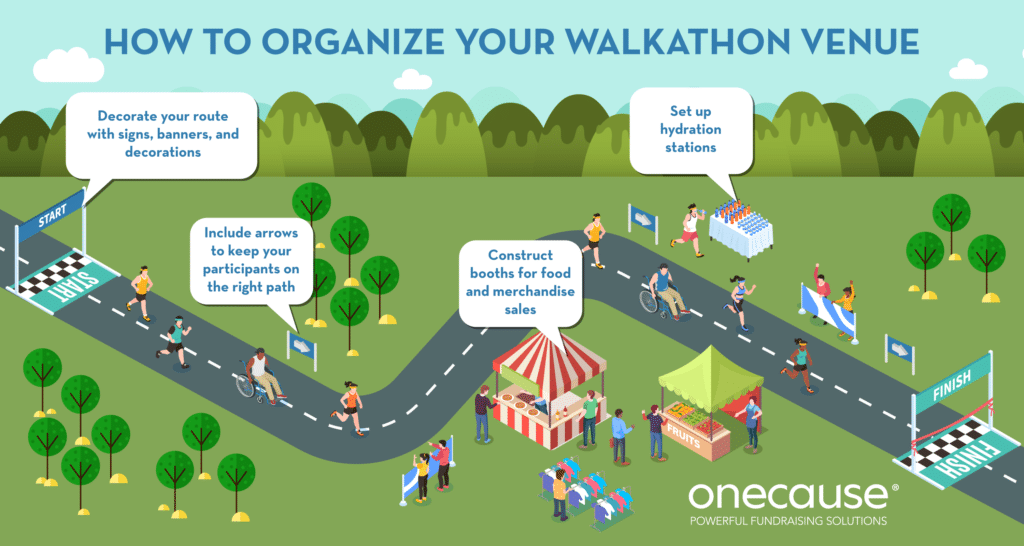This vibrant and whimsical informational poster titled "How to Organize Your Walkathon Venue" features a detailed, illustrated race path that stretches from left to right, bordered by a lush park setting with green grass and trees underneath a blue sky. The route is populated with enthusiastic walkers, runners, and wheelchair participants making their way from a clearly marked starting line to a celebratory finish line. On either side of the path, festive vendor tents for food and merchandise sales are set up, accompanied by hydration stations to keep participants refreshed. Spectators stand behind barriers, cheering on the participants. Throughout the road, helpful tips are displayed in talk bubbles including: "Decorate your route with signs, banners, and decorations," "Include arrows to keep your participants on the right path," "Construct booths for food and merchandise sales," and "Set up hydration stations." The bottom right corner of the poster features the tagline "One Cause Powerful Fundraising Solutions" in white font, indicating the sponsor of this beautifully rendered, yet simplistic digital artwork.